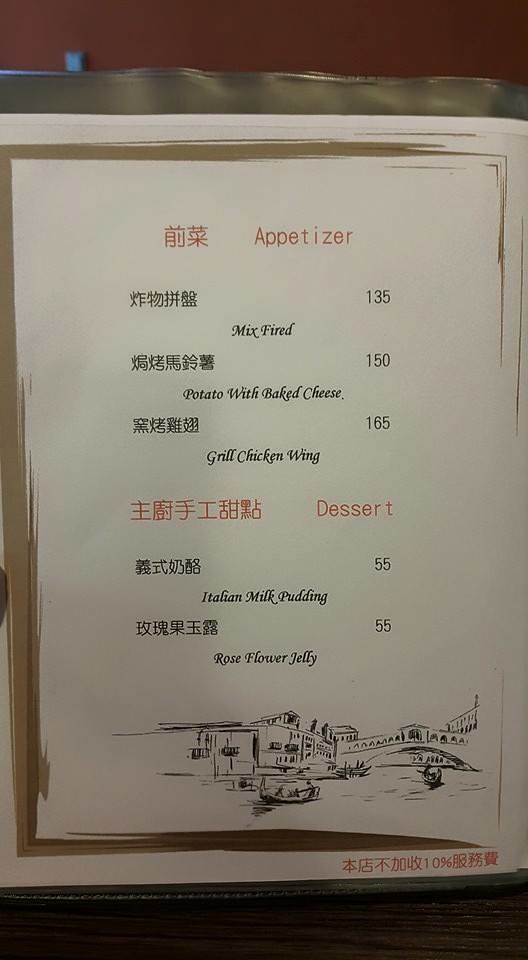This detailed caption is as follows:

"The photograph showcases a restaurant menu presented in both Traditional Chinese characters and the English alphabet. At the top, the section is labeled 'Appetizer' accompanied by its Chinese translation. Listed underneath are several appetizer options: 'Mixed Fried,' priced at 135 (currency not specified), followed by 'Potato with Baked Cheese' at 150, and 'Grilled Chicken Wing' priced at 165. 

A distinct break marked by red text introduces the next section titled 'Dessert.' The dessert offerings include 'Italian Milk Pudding' and 'Rose Flower Jelly,' both priced at 55. 

The lower portion of the menu features a hand-drawn illustration, seemingly representing a scenic view of Venice or another quintessential Italian landscape, adding an artistic touch to the menu's design aesthetic."